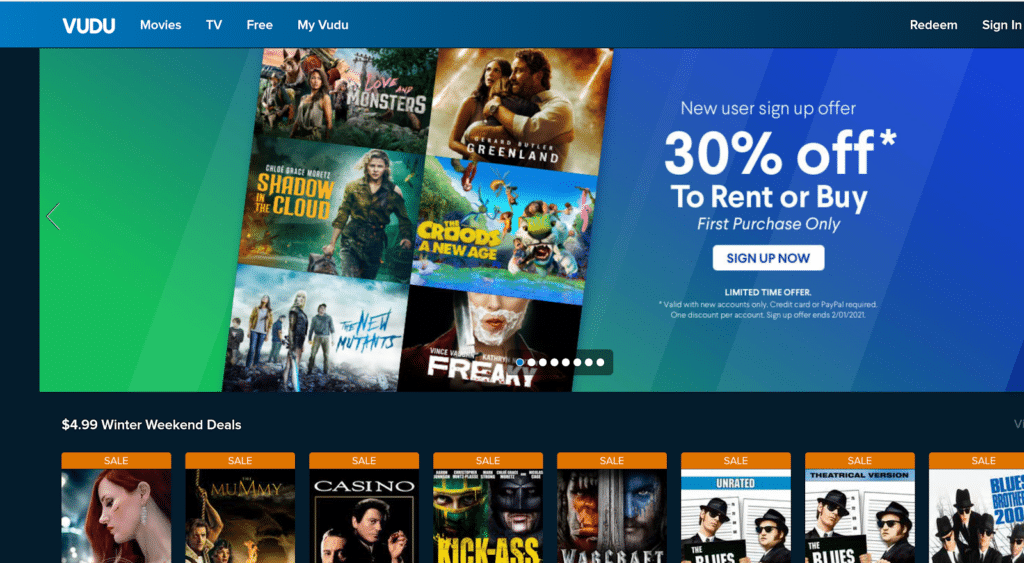The image, captured in landscape format and in vibrant color, depicts an online advertisement for VUDU, a streaming service. The central focus is the prominent VUDU logo, displayed in all caps with white lettering against a gradient banner background that transitions from light blue on the left to dark blue on the right. Dominating the middle section of the image is a bold headline reading, "NEW USER SIGN-UP OFFER: 30% OFF to rent or buy first purchase only." This suggests an enticing first-time discount for new users, though it remains unclear whether the purchase options include streaming online or physical mail delivery.

The image also showcases an array of movie thumbnails beneath the promotional text, featuring titles such as "Shadow in the Cloud" and "Greenland" among others, hinting at the diverse selection available on the platform. At the bottom of the screen, a section highlights 'Winter Weekend Deals' priced at $4.99 each, with featured films like "The Mummy," "Casino," and "Kick-Ass" displayed in a row, adding further appeal to potential customers.